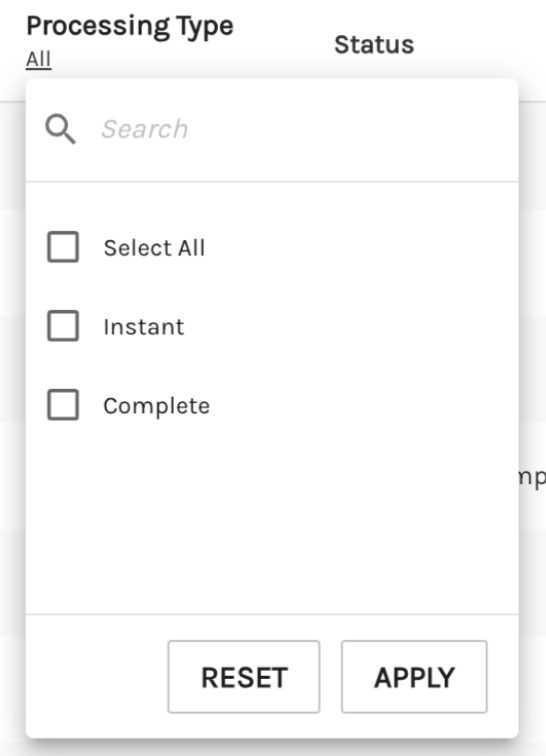The image is a detailed screenshot of a user interface window displaying a pop-up box superimposed on a larger screen behind it. The screen in the background shows a section titled "Processing Type" at the top, with the option "All" selected. To the right of "All" is a larger text reading "Status," and further down the screen, partially obscured by the pop-up, the letters "MP" can be seen against a light gray background.

The pop-up box itself is off-white in color, rectangular, and occupies almost the entire image. The top portion of the pop-up box features a horizontal section with a magnifying glass icon to the left and a grayed-out, italicized word "search" to the right, indicating a search function. Below this search bar are three vertically arranged options: "Select All," "Instant," and "Complete," each accompanied by an unchecked square checkbox to the left. There is a noticeable gap below these options, followed by a light gray horizontal line. The bottom section of the pop-up box contains two large buttons labeled "Reset" and "Apply."